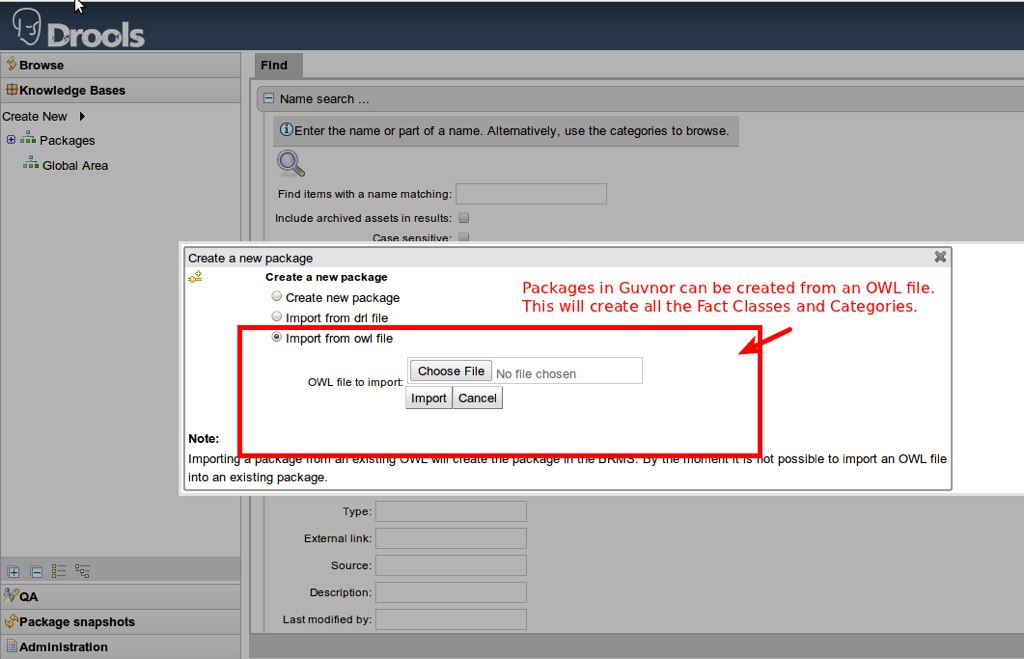The image displays a screenshot of a computer screen running a web application called Drools, identified by its name in a dark blue bar at the top left. The screenshot primarily focuses on a pop-up window with the title "Create New Package," offering options to create a new package, import from a DLR file, or import from an OWL file. The option to import from an OWL file is highlighted with a red rectangular border. Accompanying this highlight, red text reads: "Packages in Governor can be created from an OWL file. This will create all the fact classes and categories." The pop-up window includes buttons for 'Choose File,' 'Import,' and 'Cancel,' guiding the user on how and where to upload their desired OWL file. The left pane and center pane of the application's typical user interface are also visible, further contextualizing the screenshot within a tutorial or instructional framework.